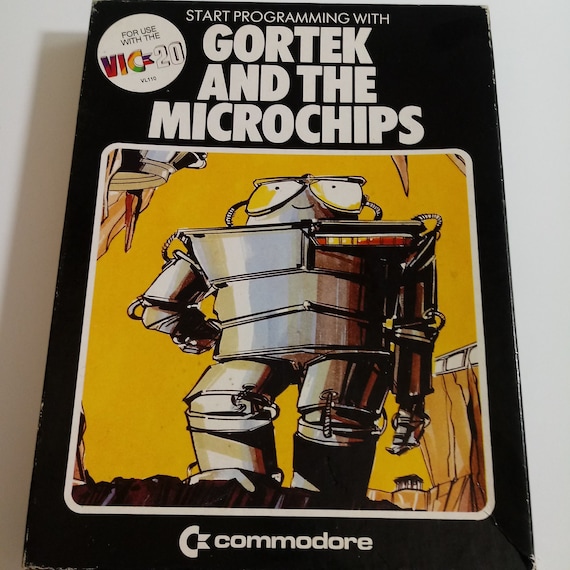The image depicts the cover of a manual or textbook titled "Start Programming with GORE-TEX and the Microchips" written in large, white, all-capital letters against a black background. The cover features a striking illustration of a humanoid, wide-built robot wearing sunglasses and posing confidently with one hand on its hip, set against a yellow backdrop. A white sticker at the top left indicates that the manual is "for use with the VIC-20," a reference to the Commodore personal computer. The word "Commodore" along with its iconic logo is prominently displayed at the bottom of the cover in white font. The detailed and vivid illustration aims to capture the reader’s attention, promising guidance on programming with the mentioned technologies.